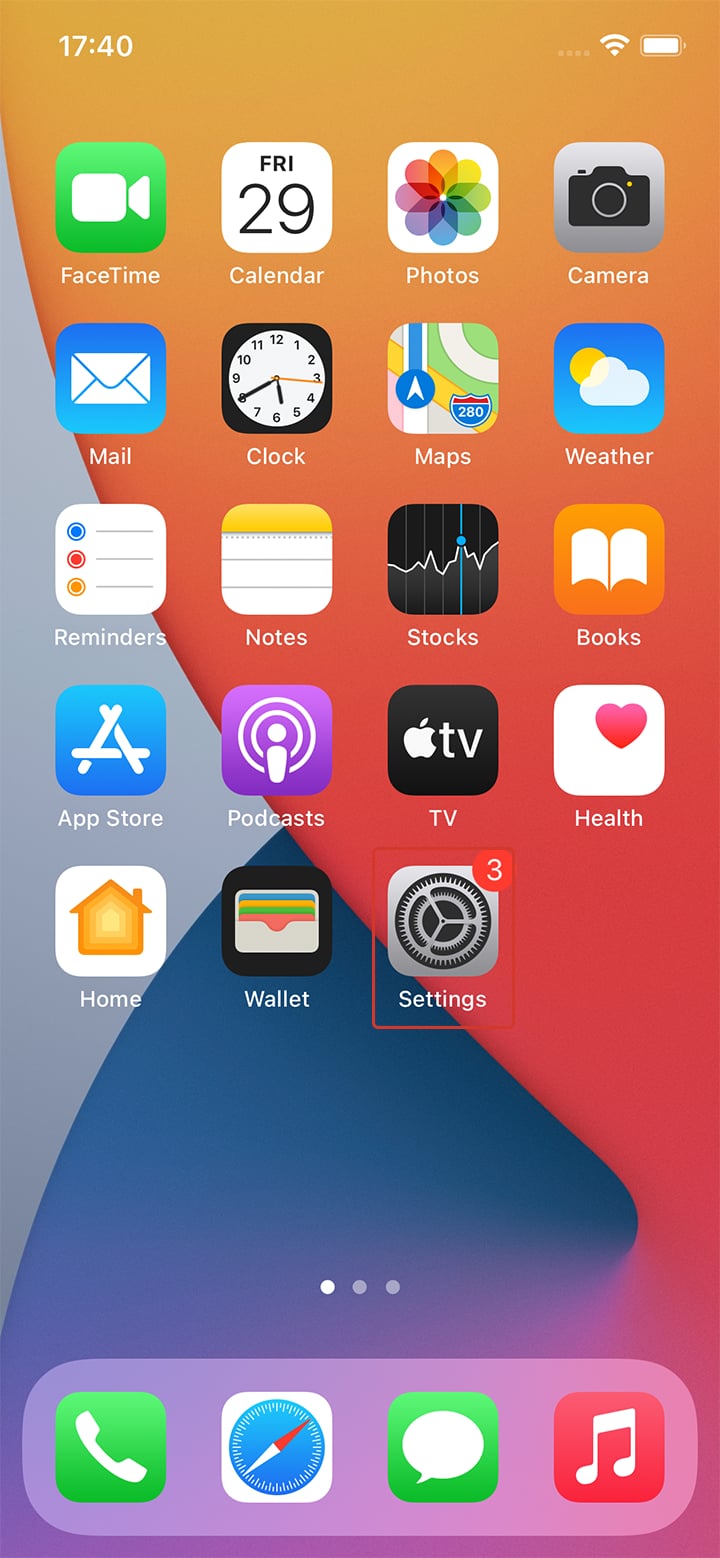A screenshot of an iPhone home page with a vibrant geometric background featuring colorful shapes in shades of orange, gray, and blue. At the very top left corner, the display shows a 24-hour clock, followed by service bars, Wi-Fi signal bars, and a fully charged battery indicator. The home screen contains five rows of apps:

1. **FaceTime, Calendar, Photos, Camera**
2. **Mail, Clock, Maps, Weather**
3. **Reminders, Notes, Stocks, Books**
4. **App Store, Podcasts, Apple TV, Health**
5. **Home, Wallet, Settings**

The Settings app stands out with a red notification badge indicating three pending alerts. Below the app grid, three dots suggest there are additional home screen pages available for swipe navigation. The bottom dock, highlighted in pink, houses the essential apps: Phone, Safari, Messages, and Music.